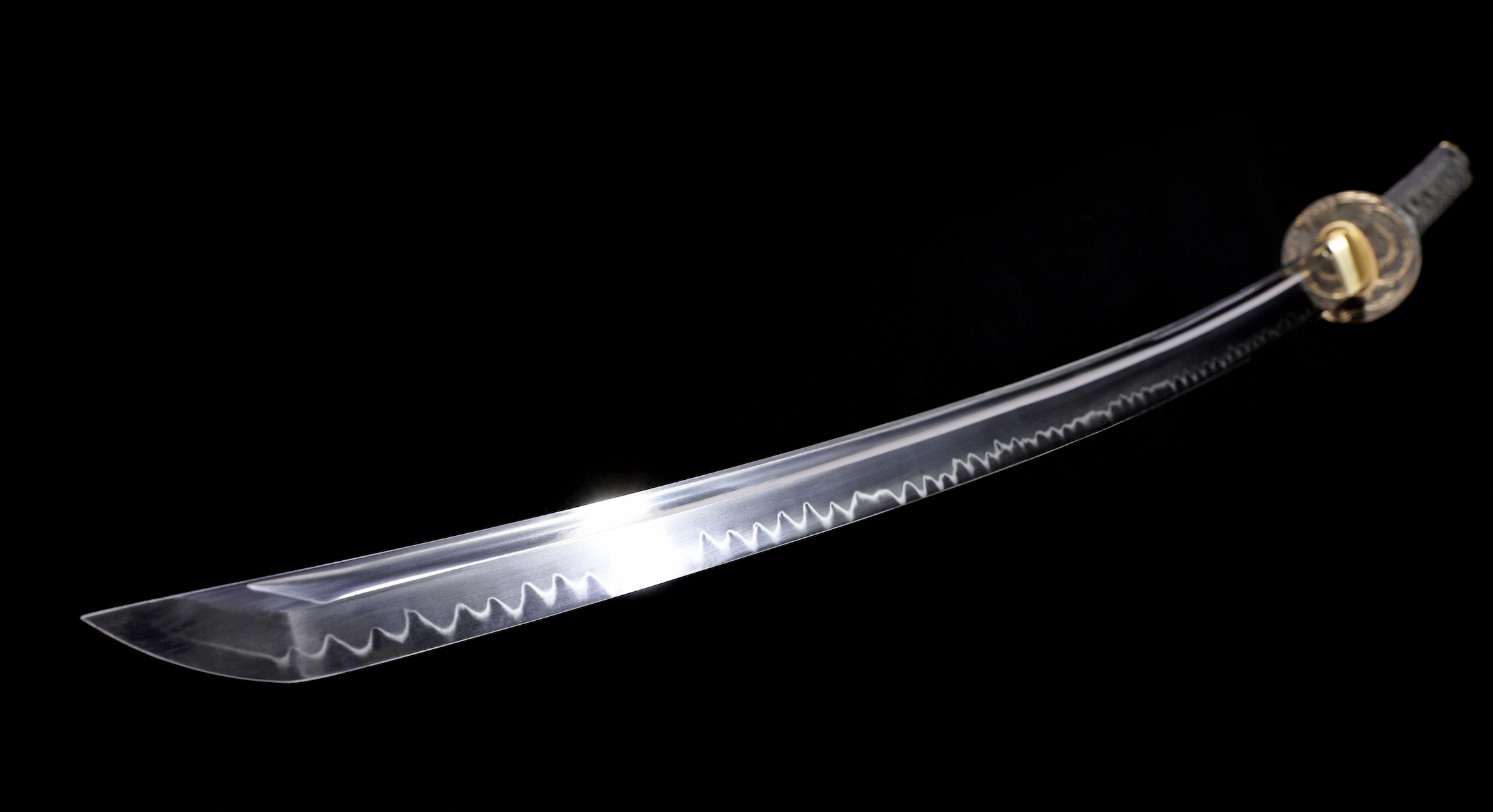The image depicts a three-dimensional digital rendering of a katana, angled at 45 degrees with the tip positioned in the lower left corner and the handle in the upper right corner. The solid black background emphasizes the sleekness and elegance of the sword, which features a silver blade reflecting light about a quarter of the way up from the tip. The blade exhibits a distinctive wavy pattern along its edge, characteristic of traditional Japanese sword craftsmanship, demarcating the sharp edge from the rest of the blade. There is a small area at the tip that appears discolored, possibly indicating an old stain. The handle is adorned with a gold round disc at the hilt, transitioning to a black grip, enhancing the weapon's intricate design and historical authenticity.